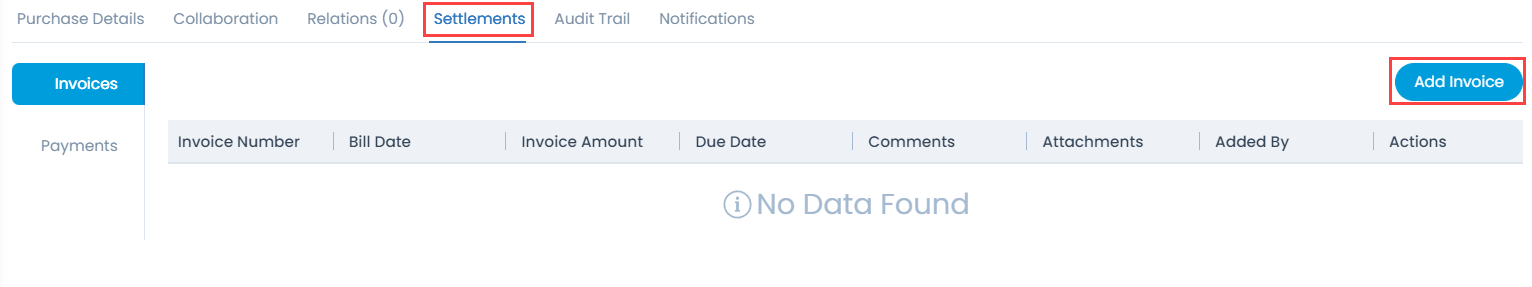The image depicts a plain, predominantly white interface. At the top, there are several tabs organized in a row. Starting from the left, the tabs include "Purchase Details" in gray, "Collaboration," "Relations" with a zero in parentheses beside it, and "Settlements," which is highlighted in blue with a red box around it. "Audit Trail" and "Notifications" follow, both in gray.

Directly beneath these tabs, on the left, there's a blue button labeled "Invoices." On the far right of this row, there's another blue button labeled "Add Invoice," also encased in a red box. 

Moving further down, there is another row that begins with "Payments" on the left. The space below this section shows various columns titled: "Invoice Number," "Bill Date," "Invoice Amount," "Due Date," "Comments," "Attachments," "Added By," and "Actions." However, at present, this table displays the message "No data found," indicating that no information is available in these columns.

The overall visual presentation is simple, with minimal color, predominantly white background and occasional accents of blue and red, drawing attention to specific buttons and links.